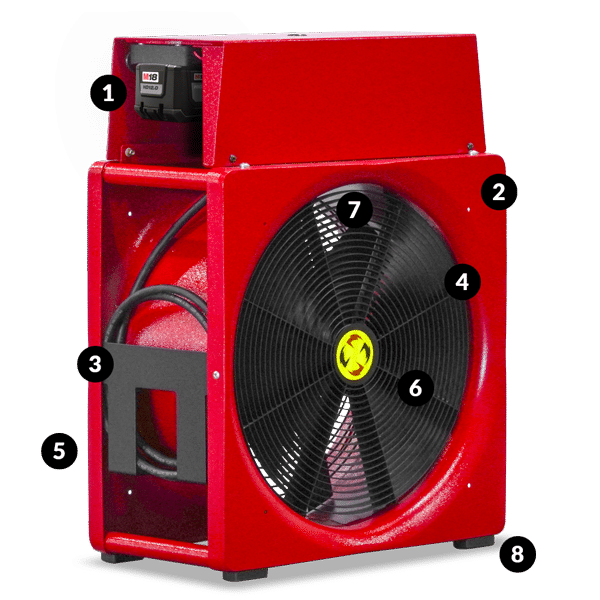The image depicts a tall and narrow red mechanical device that resembles a heavy-duty shop fan. The device features a prominent black exhaust fan on its broad, central side, which is adorned with a yellow symbol likely representing the manufacturer's logo. The fan is encircled by numbers ranging from 1 to 8 in black circles with white numerals, suggesting various functional features or adjustment levels. The shell of the device is a shiny, metallic red, giving it a distinctive appearance. Attached to the side is a black hose neatly wound up, and there are visible power cords and a handle, possibly for mobility. The device stands on three visible leg feet, indicating a stable base, with a fourth leg hidden from view. The overall construction appears durable, suggesting it is designed for industrial or heavy-duty use.